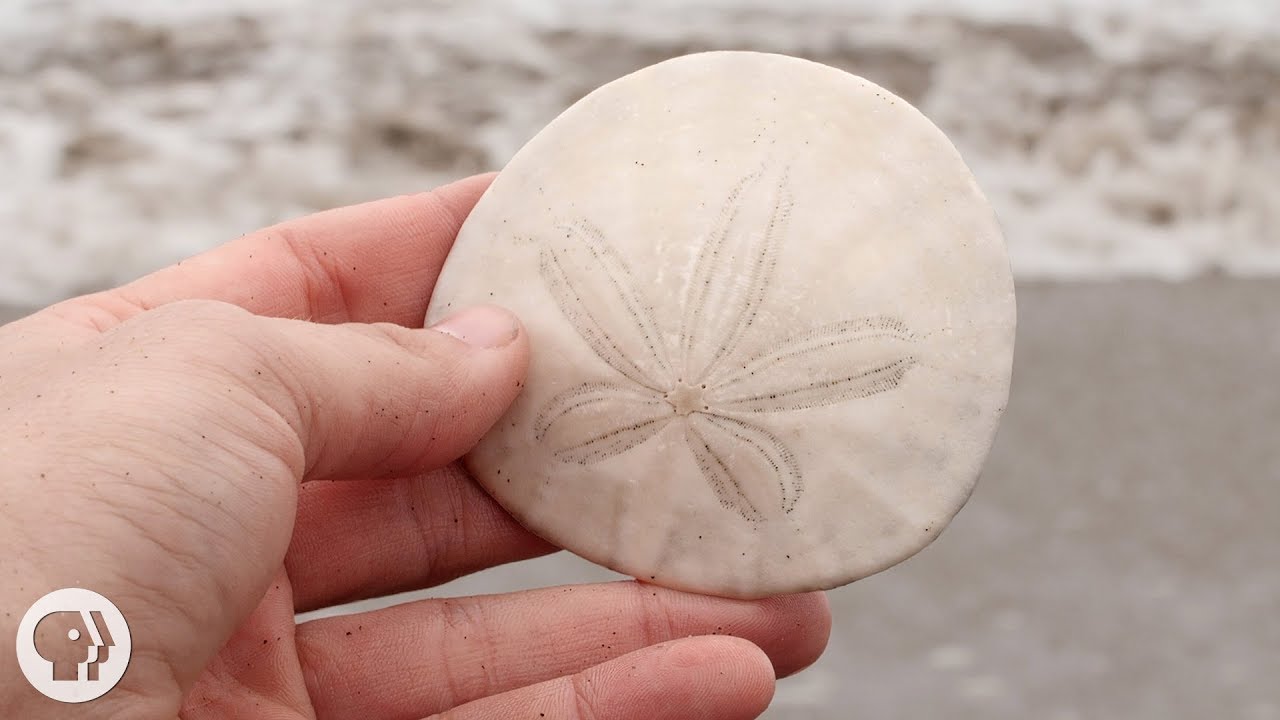In the image, a real Caucasian left hand is holding a large sand dollar, roughly the size of a palm. The sand dollar is white and features the typical five-petaled design with a star-like figure in the middle, resembling a five-leaf plant with two leaves going upwards, two downwards, and one leaf sticking straight up. The background is blurry but shows elements of the beach, with tan sand and grayish, possibly cloudy skies indicating daylight. The ocean is visible in the background with some white waves. In the bottom left corner of the image, there's a white PBS logo, which consists of a circle with the silhouette of a person's face looking to the right, and another face underneath it.